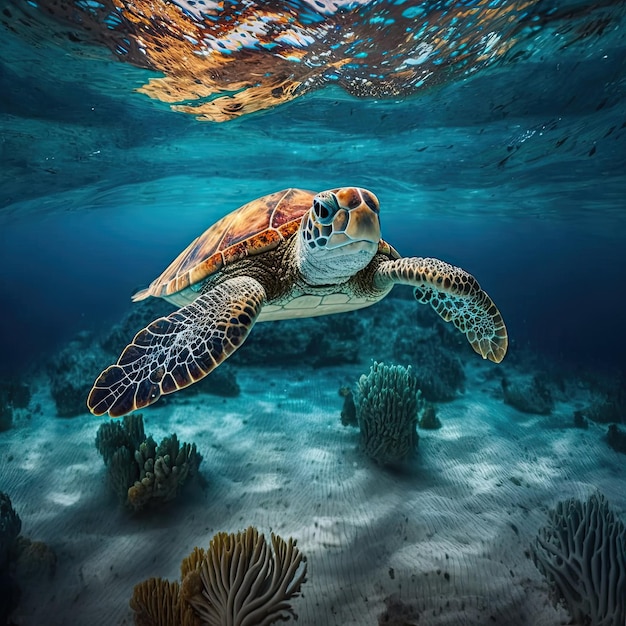This detailed, underwater painting depicts a majestic sea turtle gracefully swimming toward the viewer. The turtle, characterized by its brown, streaked shell and scaly, dark grey front flippers outlined in lighter yellowish-brown, takes center stage in the image. Its head, extending out of the shell, is painted in a vivid orange hue with blue eyelids and a black eye, gazing directly at the viewer. The turtle’s mouth is closed as it serenely navigates through the water. The backdrop reveals a shallow marine setting, with sunlight penetrating the surface and casting an ethereal glow on the turtle and the blue water around. Below, the sandy ocean floor is dotted with low-lying green aquatic plants and rocks. The upper portion of the image captures the water's surface, with an enchanting blend of orange and blue, reflecting sunlight and the turtle's presence. The overall style resembles that of a painting, enhancing the vivid detail and tranquil mood of the underwater scene.